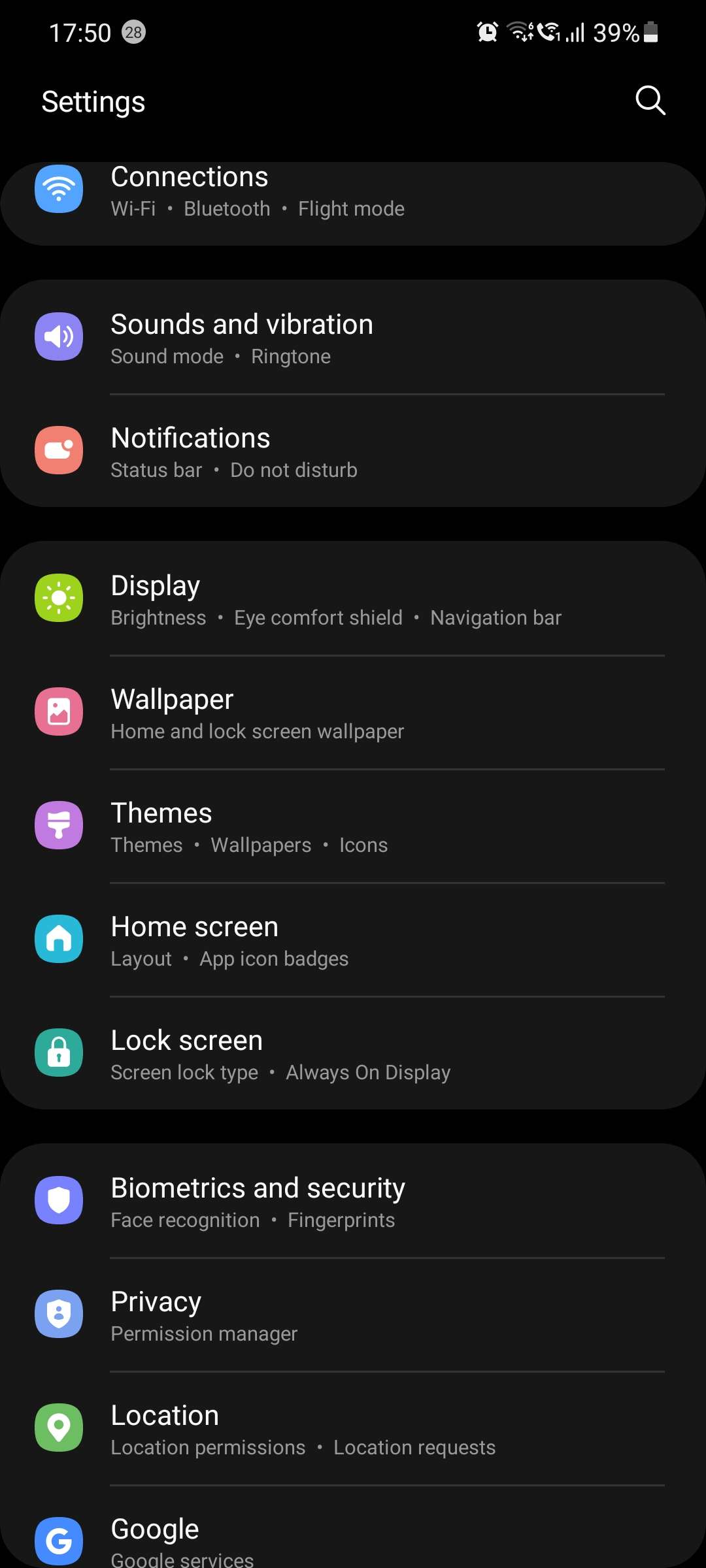This image is a vertical, rectangular display, approximately twice as tall as it is wide, featuring a black background with a list of various options, each accompanied by a distinct colored logo. At the very top left, the display shows the time, "17:50." Beneath this, "Settings" is written in white letters.

- The first entry features a blue logo with white curved lines, labeled "Connections" in white text. Below "Connections," a description reads: "Wi-Fi, Bluetooth, and flight mode."
- The second entry showcases a purple logo with a white portion depicting a volume icon, labeled "Sounds and Vibration" in white text.
- The third entry has an orange logo with a white square in the center, labeled "Notifications" in white text.
- The fourth entry displays a lime-green logo with a white sunburst in the middle, labeled "Display" in white text.
- The fifth entry presents a pink logo with a white and pink drawing resembling a landscape, labeled "Wallpaper" in white text.
- The sixth entry includes a purple logo with white elements in the center, labeled "Themes" in white text.
- The seventh entry features an aquamarine blue logo with a white house, labeled "Home Screen" in white text.
- The eighth entry is a muted green with a white lock icon, labeled "Lock Screen" in white text.
- The ninth entry displays a purple logo with a white shield figure, labeled "Biometrics and Security" in white text.
- The tenth entry has a pale blue logo with a white and blue image in the center, labeled "Privacy" in white text.
- The eleventh entry shows a green logo with white and green elements, labeled "Location" in white text.
- The twelfth and final entry presents a blue icon with a white capital "G" in the center, labeled "Google" in white text.

At the upper-right corner of the rectangle, small icons are visible alongside a magnifying glass symbol, representing a search function similar to online search bars.